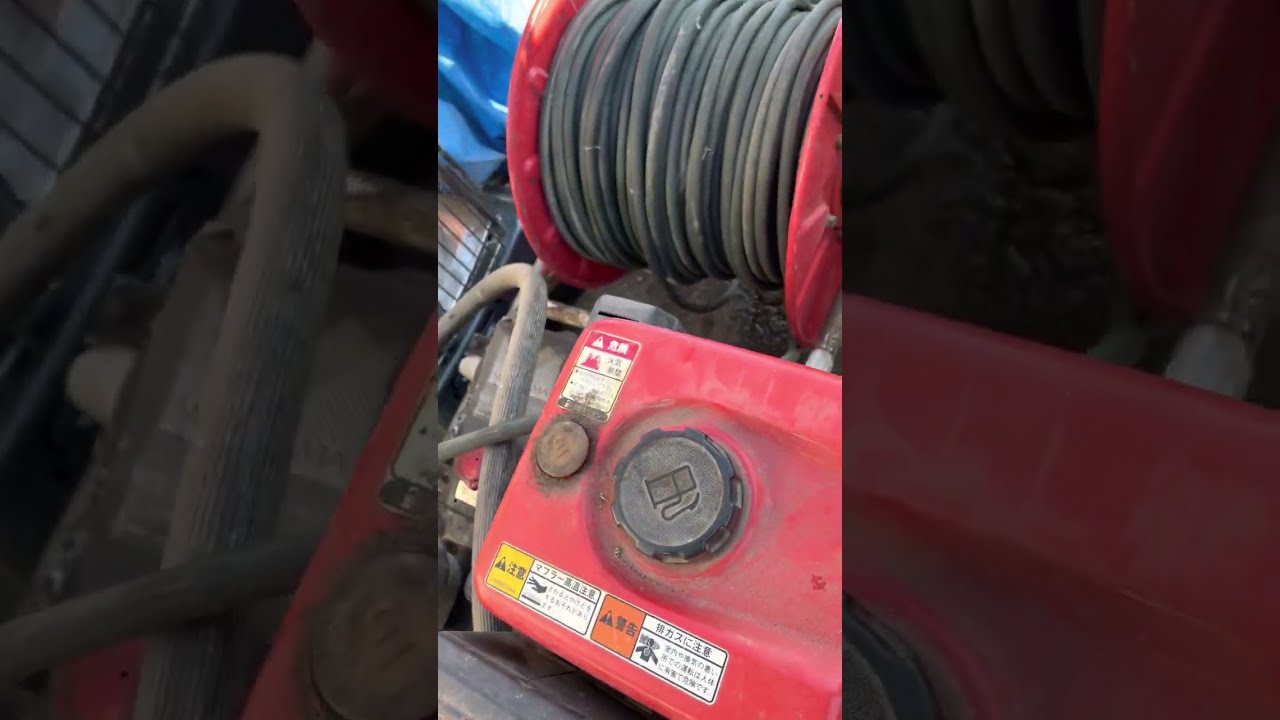The image showcases a construction or workshop scene centered around a gas-powered generator and a heavy-duty spool. The red generator occupies the bottom half of the image and features prominent yellow, white, and orange warning labels in a non-English language, suggesting an international make. The generator is topped with a blue cap, adorned with a gas pump logo, and detailed grooves for easy grip. Directly above the generator, a large, red spool with black heavy-duty rope is prominent, indicating equipment used for heavy lifting or wiring. In the top-left corner, a blue object that might be a tarp can be seen. The entire scene appears to be framed, possibly simulating a social media post or a video screenshot, emphasizing a workspace environment.